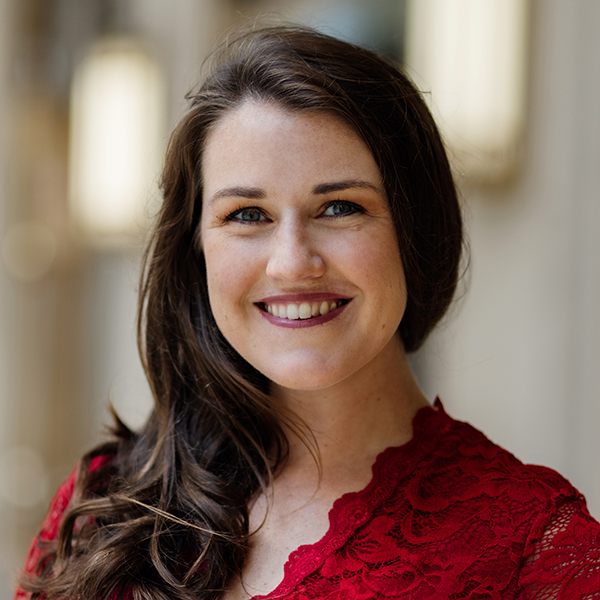This photograph appears to be a LinkedIn profile picture of a woman with fair skin, brunette hair, and striking blue-green eyes. She is smiling brightly, revealing her top teeth, and giving off a very warm and happy aura. Dressed in a red lace dress with a V-shaped neckline, her long, curled hair cascades elegantly over her right shoulder. The photo is tightly framed, focusing on her head and cutting off just below her shoulders, making it a classic headshot. The background is blurred and light-toned, ensuring that the attention remains on her. She is not wearing any jewelry, and her mauve lipstick complements her polished look. The overall impression is one of a professional, yet approachable and classy individual.